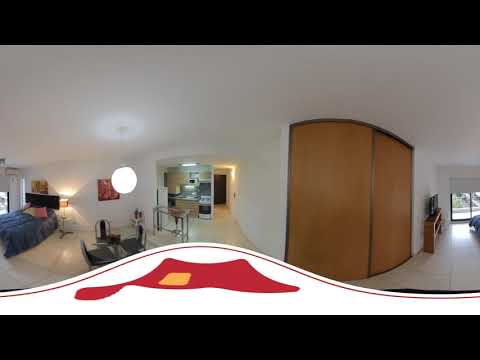This detailed interior photograph, likely taken inside a house, captures a panoramic view of a room with predominantly white walls and ceiling. On the left side, there is a bed featuring a blue mattress adorned with pillows, primarily pink and yellow in color, beside which stands a bright white lamp. Adjacent to the bed is a window, bringing natural light into the space. To the right of the bed, there is a cozy setup with three small black chairs surrounding a white light fixture that hangs from the ceiling. 

This seating area also includes a small table and is positioned near an open area leading into a kitchen, identified through a squared archway. The kitchen area features some visible appliances and a partial table, enhancing the residential feel. Further right, there is either a sliding door or large drapes concealing a big window or entrance, which might connect to a hallway.

To the far right, the room extends to a wooden bookshelf or shelf area, situated next to a large double-door closet. The floor, like the rest of the room, is white, possibly polished tile. No people are present in the image, and despite the evident daylight, the lamps in the room are illuminated, adding a warm ambiance to the airy, white-themed space.